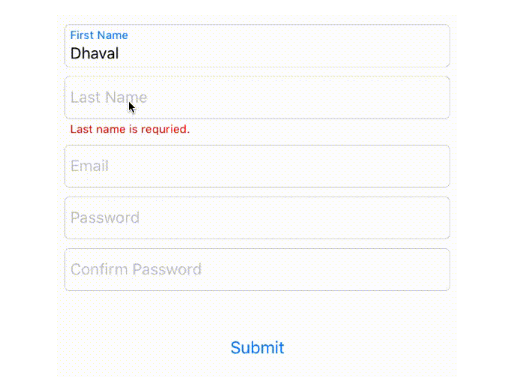A partial screenshot displays a minimalist signup form, possibly from either a smartphone or a computer, with no visible header or footer to provide contextual clues. The background of the form is a clean white, enhancing the clarity of the five outlined rectangular fields presented. 

The topmost field prominently features the label "First Name" in blue font, with the user input "DHAVAL" displayed beneath it in black. Following this, a gray-labeled "Last Name" field is conspicuously highlighted by a red error message stating "Last name is required", accompanied by a small black arrow pointing to the field, indicating the need for correction. 

Subsequent fields are designated for "Email", "Password", and "Confirm Password", maintaining the same gray outline for uniformity. Central at the bottom of the form, the "Submit" button is attractively presented in blue font against the white backdrop, inviting the user to finalize the creation of their account.